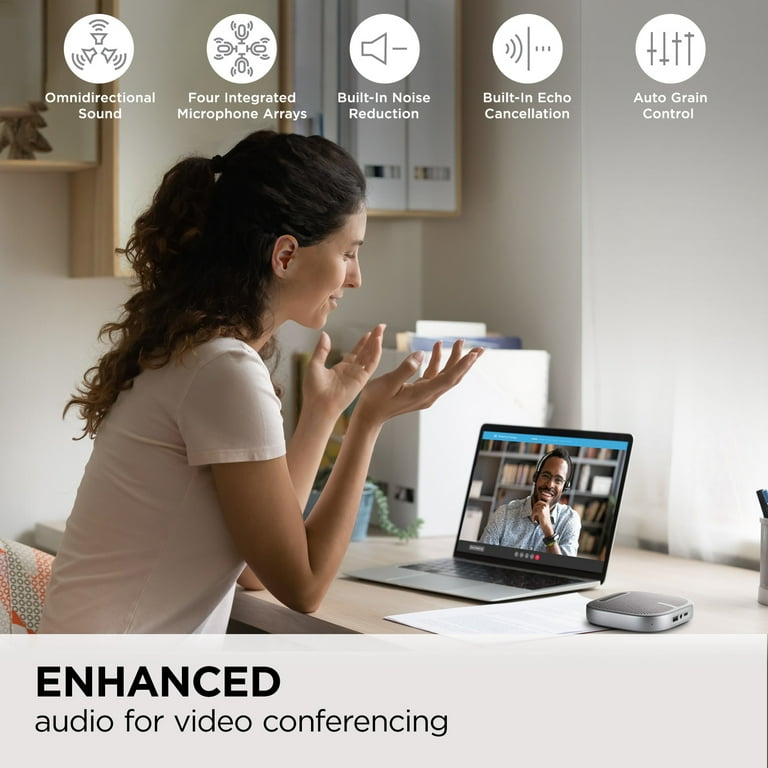This is an advertisement poster featuring a central image of a woman engaged in a video conference. At the top of the poster are five white circles with simplistic grey illustrations, each accompanied by a label detailing specific audio features: Omnidirectional Sound, Four Integrated Microphone Arrays, Built-in Noise Reduction, Built-in Echo Cancellation, and Auto Gain Control.

In the main image, a young woman, likely in her thirties, sits at a desk or counter with a laptop in front of her. She has long dark hair tied back in a ponytail and is dressed in a white short-sleeved shirt. She faces to the right, looking down slightly, with both of her hands raised palms up. On the laptop screen, she is in a video call with a man who has earphones on. He is smiling and has his hand up to his chin, dressed in a light blue long-sleeved collared shirt. The room’s background is primarily white, showing some shelves.

At the bottom left of the poster, there is a grey border featuring bold black text that reads "ENHANCED" and below, in smaller black text, "Audio for Video Conferencing."